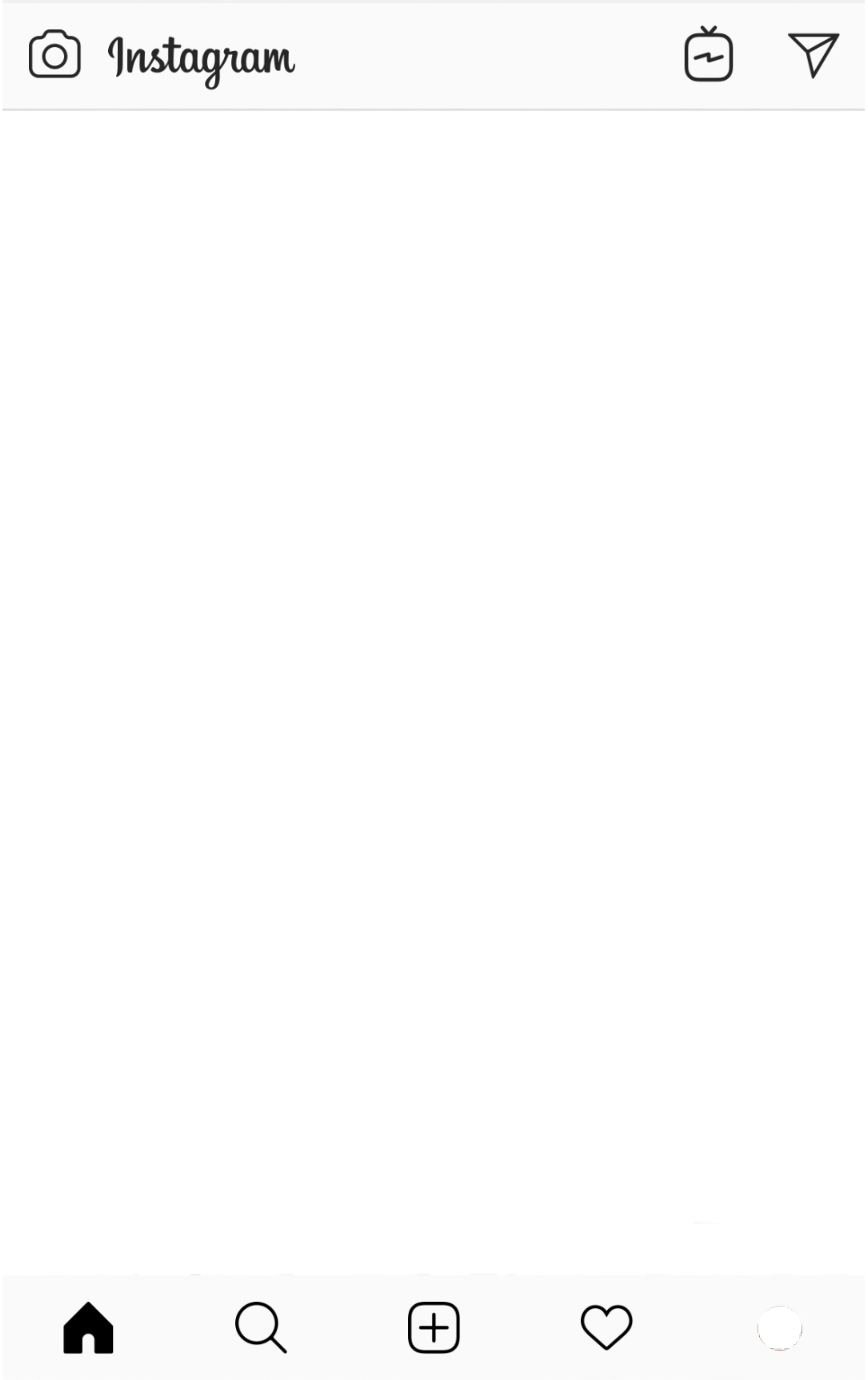Screenshot of a Blank Instagram Interface

This image is a screenshot capturing a blank Instagram interface, indicating a potential app malfunction or lack of data retrieval. The top section prominently features the Instagram logo, accompanied by a direct message icon represented by a paper plane image, and a TV icon likely for Instagram Reels or IGTV. Below this header, the screen is entirely white, signifying no content is being displayed. 

At the bottom, the standard navigation bar is visible, displaying the home button, search function, create button, activity (likes or favorites), and the user profile. The empty middle part of the screen is where posts, stories, and other content typically appear, but here it sits vacant, suggesting the user encountered an issue with loading content. 

This screenshot effectively highlights an instance where Instagram appeared unresponsive or without any displayed data, presenting a sleek and minimal user interface without any active content.